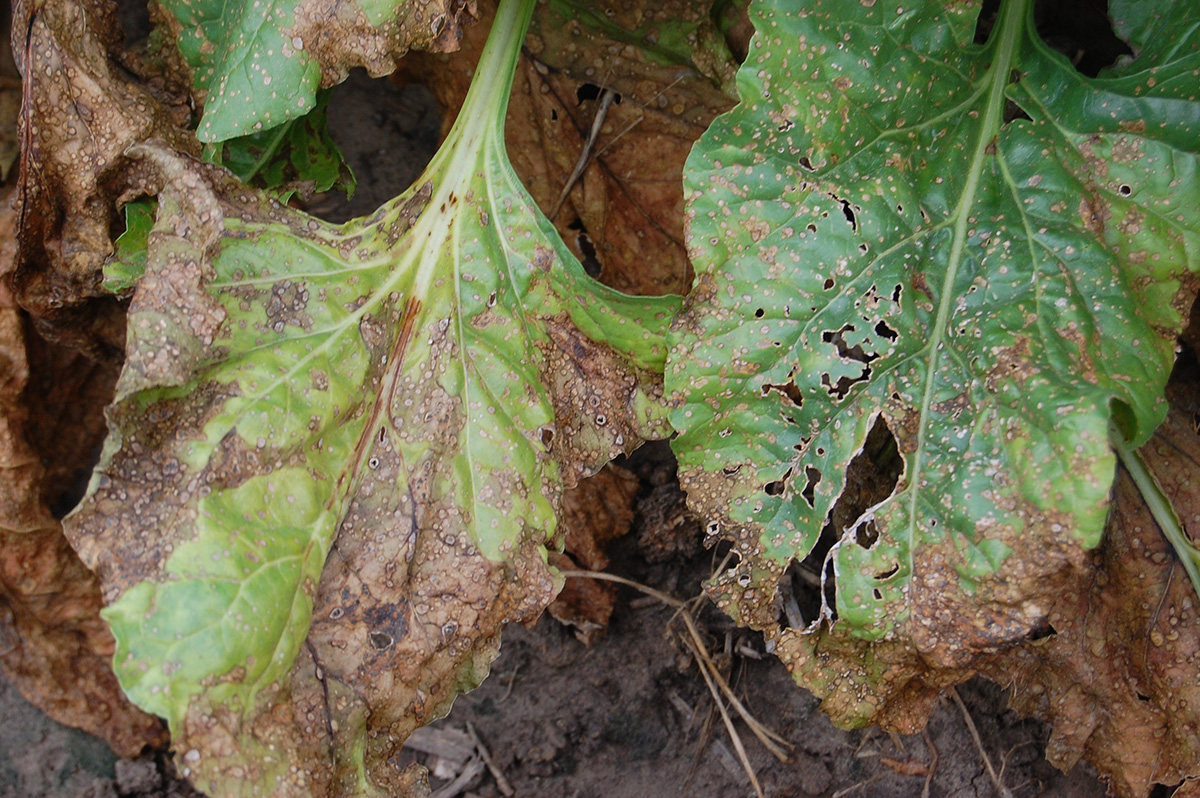This close-up photograph captures a detailed view of two prominently displayed leaves amidst a backdrop of similarly desiccated foliage. The leaves, resembling large spinach or lettuce leaves, dominate the image with their distressed appearance. Both leaves are heavily shriveled and browned, with the right leaf exhibiting noticeable holes, likely from pest activity. The left leaf shows signs of yellowing at its edges, an indication of its deteriorating condition. While the primary color of the leaves was originally green, they now display extensive brown and dry patches. The background reveals more leaves out of frame, also primarily brown and crisp, suggesting widespread rot or the effects of an autumnal decline. The ground beneath the leaves is partially visible, showing muddy and wet conditions. The photo is tightly framed, with no visible stems, flowers, or other objects.